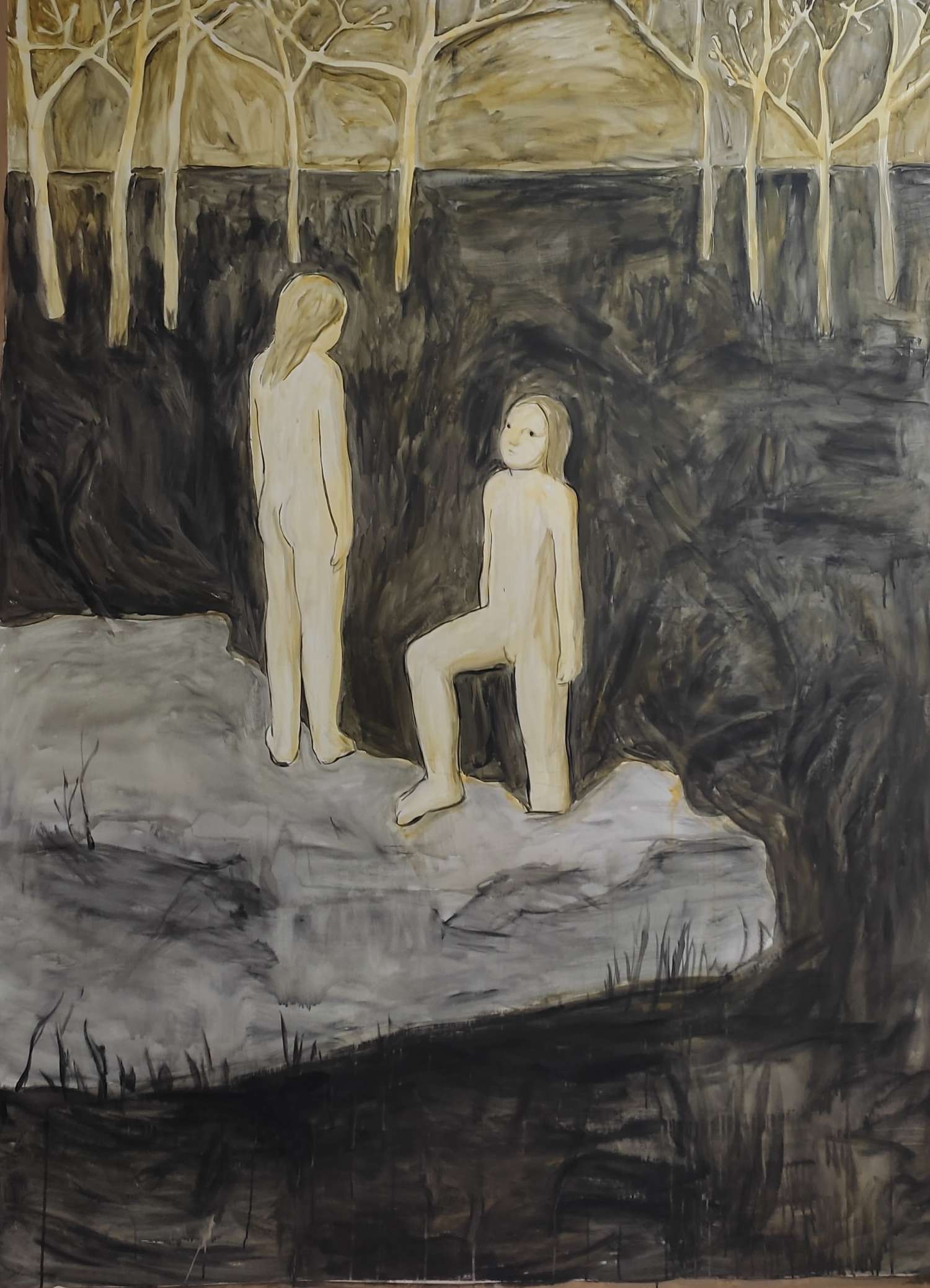The painting, a work of art rendered in acrylics with possible pencil or fine pen details, depicts two androgynous figures on a gray rock formation amidst an abstract landscape. These human-like figures, who both appear to be female, are unclothed and featureless, sharing identical skin tones and hair colors, suggesting a twin-like resemblance. The person on the right is shown climbing onto the rock from black waters below, her body positioned with one leg bent on the rock and both arms hanging loosely by her sides. The other figure is standing on the rock, facing away from the viewer, her back, arms, and legs outlined without distinct anatomical features.

Surrounding the central figures, the landscape is minimalistic, with black strokes resembling grass and distant, golden-hued trees under a beige sky, lending the scene a darker yet non-sinister atmosphere. The overall composition combines elements of abstraction and surrealism, focusing on form and movement rather than realistic detail.